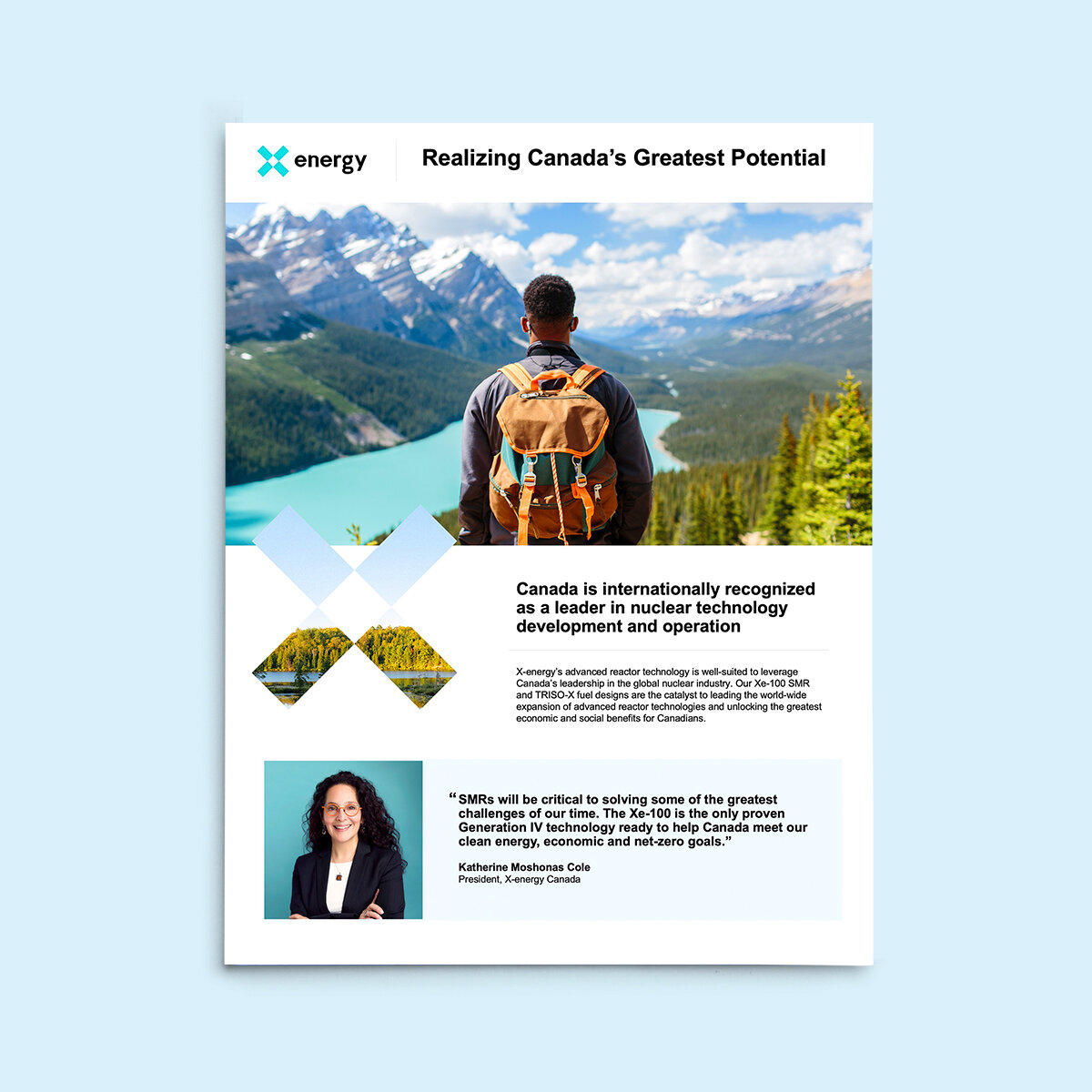**Caption:**

The image features a visually appealing advertisement that appears to be either a blog article or a promotional poster. It is meticulously designed and divided into several distinct sections.

At the top left of the image, there's a blue X icon with a white diamond in the center. To the right of this icon, the word "energy" is written in dark blue, nearly black, lowercase letters. Adjacent to it, in the same size but in title case, the text reads: "Realizing Canada's Greatest Potential." This entire header section is placed on a white rectangular bar that spans the width of the image.

Below this header is a captivating main image. It shows the back view of a person, possibly male, wearing a dark blue jacket and an orange backpack. The individual appears to be standing in a natural setting, overlooking a picturesque valley with a river running through it and mountains on either side. The sky is blue with puffy clouds, and the landscape is rich with forested areas. The sun shines brightly over the scene. The individual is dark-skinned with hair that resembles a small afro.

Upon further inspection, the bottom section of the image retains the visual branding of the top left icon; the blue X icon reappears but this time, it’s filled with an image of natural elements such as sky, forest, and lake. To the right of this icon, there's text that states: "Canada is internationally recognized as a leader in nuclear technology development and operation." Another set of smaller text exists beneath, but it is too small to read clearly.

Below this informative section, there's a highlighted area with a thumbnail image of a woman. She has black, curly hair, is wearing glasses, and is smiling at the camera while crossing her arms. She is dressed in a suit jacket and has a blue background behind her. Beside her image is a quote: "SMRs will be critical to solving some of the greatest challenges of our time. The XC 100 is the only proven Generation IV technology ready to help Canada meet our clean energy, economic, and net zero goals." The quote is attributed to Catherine (last name unclear), president of X Energy Canada.

The entire poster or article is paper-sized with a drop shadow effect, which is embedded within a larger light blue rectangle that serves as the background for the image.